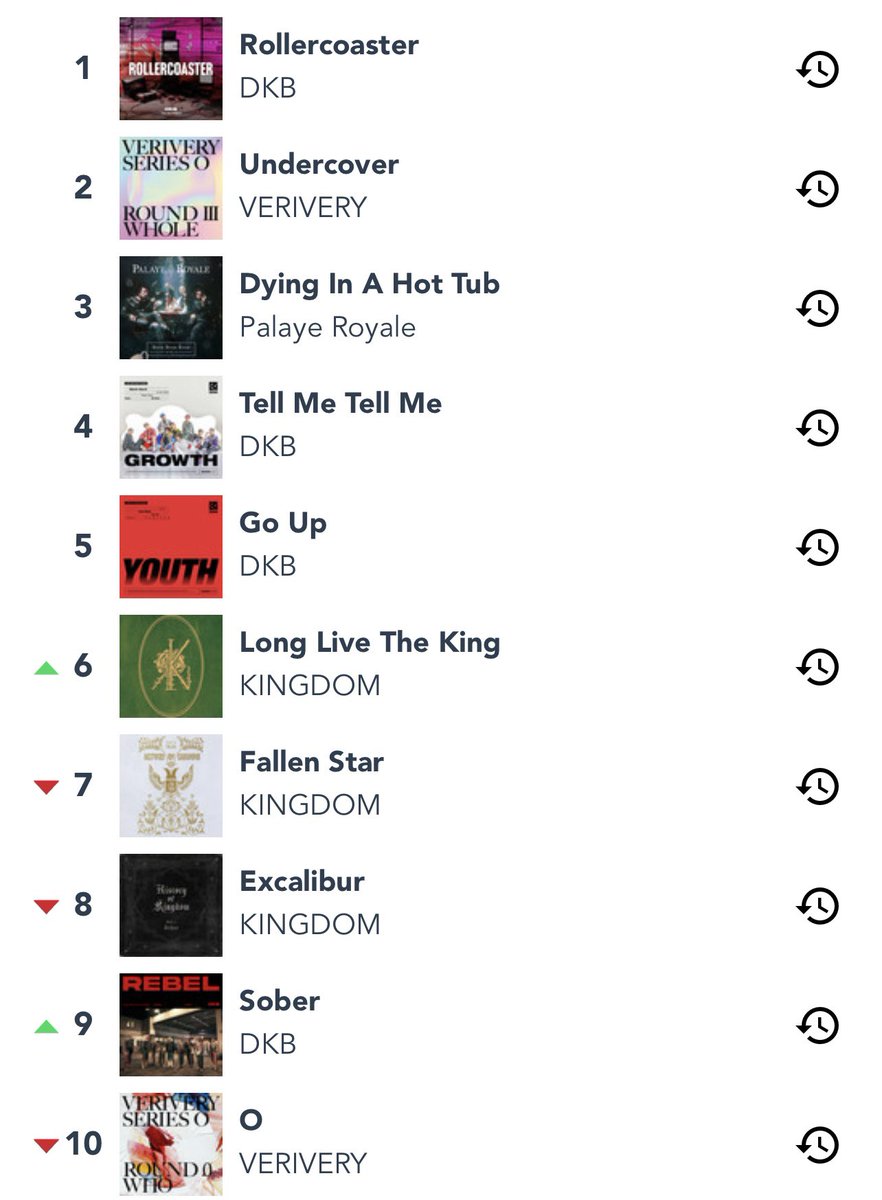Here is a cleaned up and detailed caption for the described image:

---

The image is a screenshot of a mobile phone interface displaying a ranked list of music albums or songs. The screen is in portrait orientation with a clean white background and black text. The list includes ten entries, each accompanied by descriptions and ranking indicators. 

At the top of the screen, each entry is organized with the first line of text in bold, likely indicating the title of the track or album, and the second line in regular text, possibly the artist. On the right-hand side of the screen, there is a "History" or "Recent Activity" button, symbolized by a clock icon encircled by an arrow.

The ranked items are as follows:

1. **Roller Coaster** by DKB
2. **Undercover** by Very Very
3. **Dying in a Hot Tub** by Palais Royale
4. **Tell Me Tell Me** by DKB
5. **Go Up** by DKB
6. **Long Live the King** by Kingdom (indicated with an orange triangle pointing up, suggesting a rise in rank)
7. **Fallen Star** by Kingdom (indicated with a red triangle pointing down, suggesting a fall in rank)
8. **Excalibur** by Kingdom (also marked with a red triangle pointing down, suggesting another drop in rank)
9. **Sober** by DKB (highlighted with a green triangle pointing up, suggesting an improvement in rank)
10. **Oh** by Very Very (marked with a red triangle pointing down, suggesting a decline in rank)

The neatly organized list outlines current trending tracks, with visual indicators showing changes in the ranking positions for each song.

---

This descriptive caption conveys a clear and detailed understanding of the screenshot's contents.